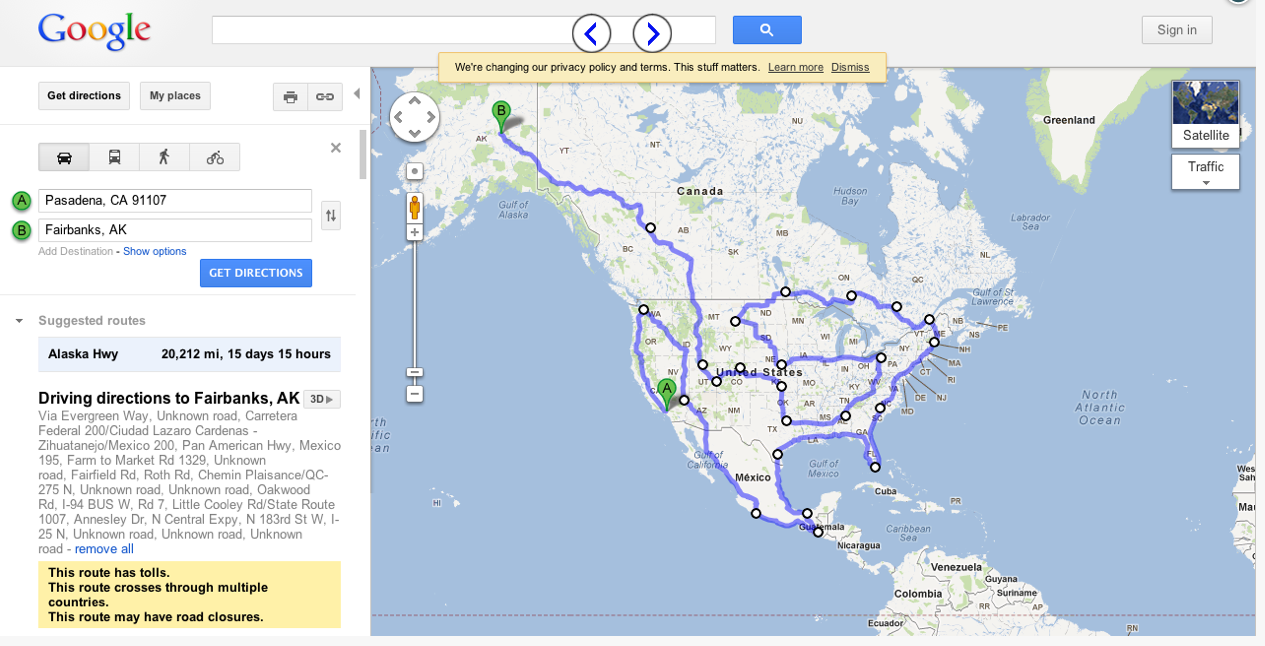This is a screenshot of a Google Maps interface taken from a desktop or laptop. The map prominently displays the United States, most of Canada, and some northern parts of South America, emphasizing a detailed route starting in Pasadena, California, and ending in Fairbanks, Alaska. The map is rectangular in shape with a light blue border at the top, where the word "Google" appears alongside a search bar. A blue tab with a magnifying glass icon is near the center of the map. The top right corner has a light white button labeled "Sign," and below it, there are options for getting directions, managing favorite places, and accessing general travel information. The displayed route is purple with circular markers indicating various cities and stop-off points. The landmass is white, and the water is light blue. The route from Pasadena to Fairbanks is marked with green 'A' and 'B' markers respectively and runs through multiple states, into Canada, and ultimately to Alaska.